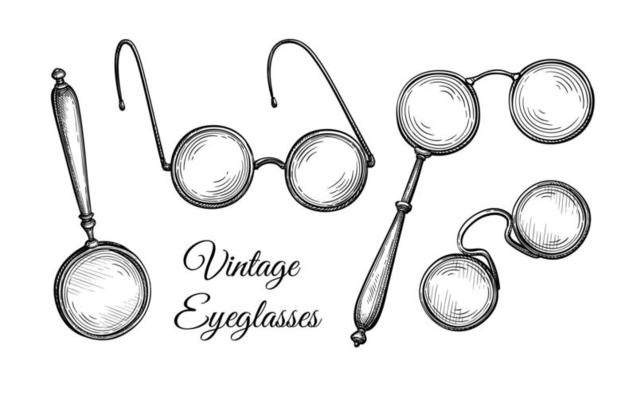This detailed black pen drawing features four distinct styles of vintage eyeglasses against a stark white background. At the bottom of the image, the words "vintage eyeglasses" are elegantly scripted in an old-fashioned cursive font. Starting from the left, the first item is a traditional magnifying glass with a prominent handle, showcasing a round, heavy lens that emphasizes its magnifying capability. Next to it, there is a pair of wireframe spectacles with a curved nose piece and ear hooks, representing the classic eyeglass design still familiar today. The third item resembles opera glasses, characterized by two round lenses connected by a nose piece and equipped with a handle, allowing them to be held up to the eyes for improved vision. Lastly, the fourth style features pince-nez glasses, designed to sit directly on the nose with a curved nose piece that loops up and over the nose, eliminating the need for ear hooks. Each of these vintage eyeglass styles is meticulously drawn, showcasing the diverse range of historical eyewear.